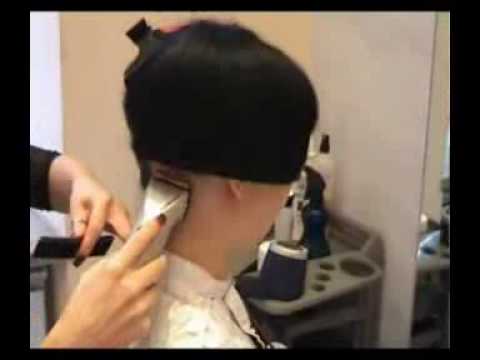In this indoor photograph taken inside a salon, a man with white skin, wearing a white shirt, is seen getting his hair cut. The back of his head, neck, and shoulders are visible as a woman with painted nails holds a silver-colored electric trimmer against the back of his neck. A ring adorns her left thumb. In her other hand, she also holds a comb. His black hair is straight and reaches mid-ear length. Visible in the background is a green wall adorned with shelves that hold various hair salon equipment including air spray and a blow dryer. To the right, a partial view of a mirror can be seen. The image is framed by a black border.